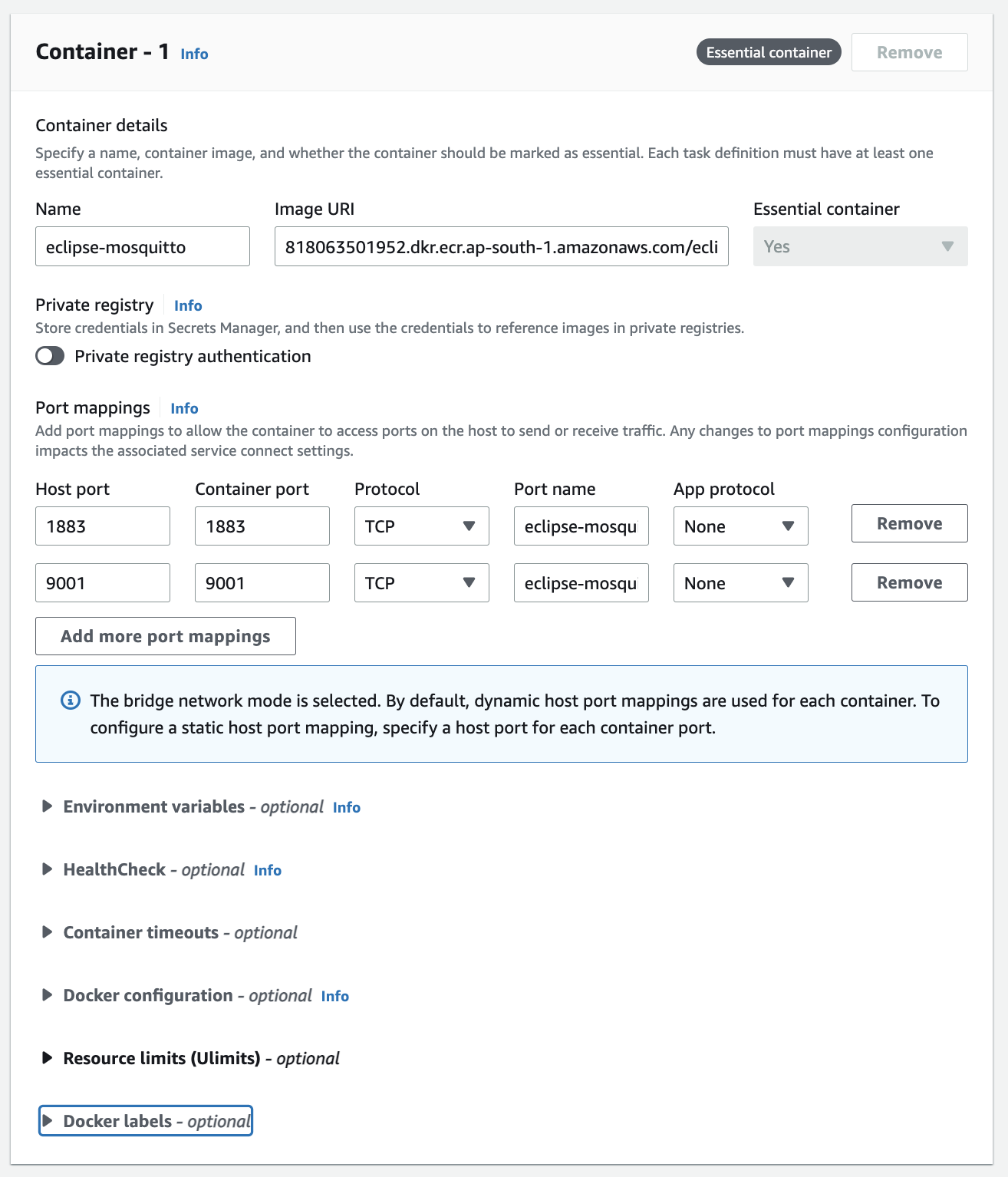The image shows a vertically rectangular screenshot taken from a slide tour application, displayed on a predominantly white background. At the top of the frame, “Container 1” is written in black text, and adjacent to it, a blue hyperlink labeled “Info” is visible. On the right side, there is a heading that reads “Essential Container,” next to a “Remove” button. Below this, the section titled "Container Details" provides form fields and instructions necessary for configuring a container.

The "Container Details" section guides the user to specify:
- **Name:** A field for typing in the container's name.
- **Container Image:** A field for typing in the image URI.
- **Essential Container:** A dropdown menu with options "Yes" or "No" to indicate if the container should be marked as essential. The instructions note that each task definition must include at least one essential container.

Further down, there is a section labeled "Private Registry," which includes another "Info" link in blue. It contains fields and options for storing credentials in the Secrets Manager and using these credentials to reference images from private registries.

The image continues down to provide configuration options for port mappings, which include:
- **Host Port:** A field for the host port number.
- **Container Port:** A field for the container port number.
- **Protocol:** A dropdown menu to select the protocol.
- **Port Name:** A field for the port name.
- **App Protocol:** Another dropdown menu to choose the application protocol.

The screenshot captures a detailed step-by-step interface for configuring container settings, with clear headings, instructions, and input fields for defining essential elements of a container setup.